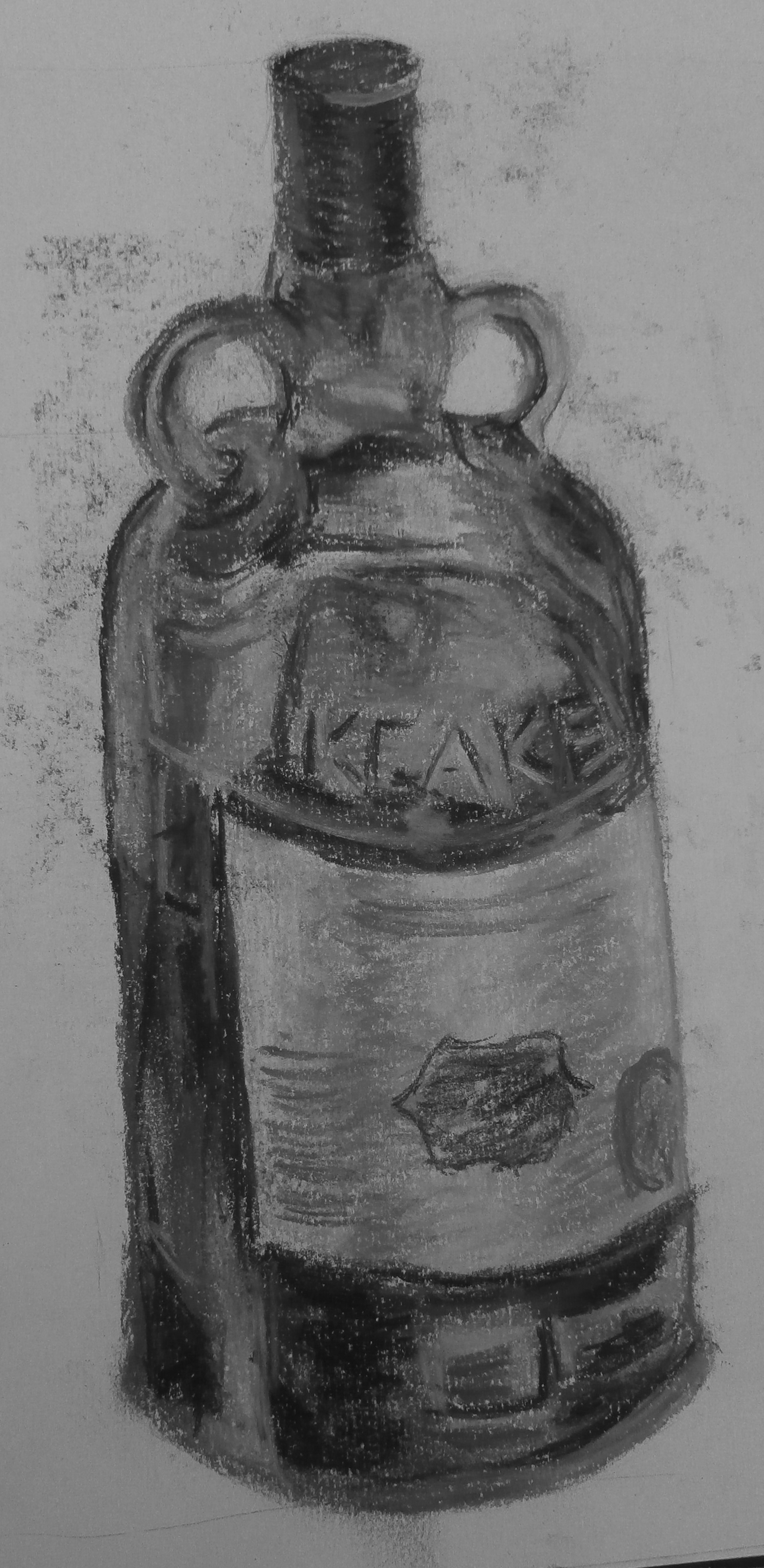This vertically tight-cropped photograph showcases an intricately detailed charcoal drawing of a vintage glass bottle, centered and slightly tilted to the left. The bottle features distinct engraving or raised detailing above a central label inscribed with the letters "I-K-E-A-K-E." Highlighted contrast between the shadows and the reflective surfaces of the glass evokes a realistic texture. The bottle is artistically illustrated with two handles or circular elements beneath the cap. Additional embellishments, including a star-shaped object and a circle, adorn the label, contributing to the drawing's overall intricate and lifelike appearance.